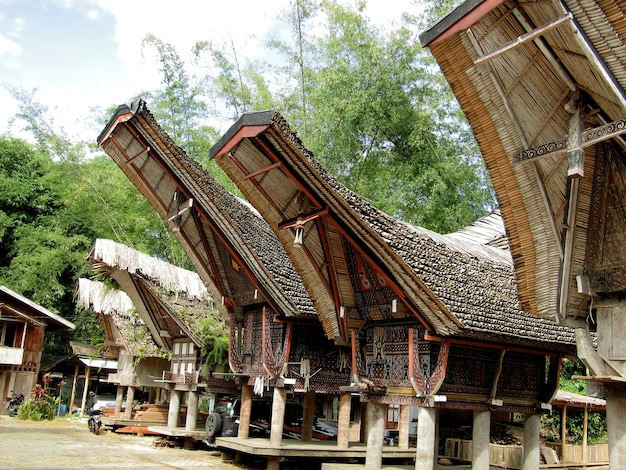This outdoor photo captures a bright daylight scene of traditional, elevated native buildings, possibly located in Asia. The structures are built on wooden platforms with stilts, raising the main part of the buildings off the ground. The roofing is distinctive, extending outward and upward at sharp angles, resembling the open mouth of a crocodile, and appears to be made of wood or bamboo. The buildings are adorned with intricate paintings or decorations. A jeep or SUV is parked beside one of the structures, hinting at modern usage, perhaps even as an Airbnb. In front, there might be fabric-covered entrances, leading to small decks. In the background, a long tree line of tall, green trees stands against a bright blue sky, dotted with white clouds.